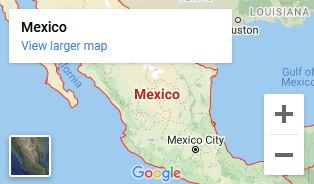A Google Maps screenshot showcasing the regions of Mexico and the southern United States. On the left side of the image, the Pacific Ocean is labeled in blue, while on the right side, the Gulf of Mexico is also labeled in blue text. In the upper left corner, a white rectangle with black text indicates "Mexico," accompanied by blue text underneath that reads "View Larger Map." In the bottom left corner, there is a detailed topographical map highlighting Mexico and the very southern parts of the United States. This map, captured most likely from aerial images, reveals grayish-white areas outlined in dark gray. In the upper right corner, the word "Louisiana" is visible, and to its left, "Houston" can be partially read, though the "H" is cut off. Near the center of the image, "Mexico" is clearly marked, with "Mexico City" positioned about a quarter down from the top. At the bottom center, the Google logo is displayed. On the right-hand side of the image, a horizontal rectangle features gray plus and minus symbols for zooming in and out of the map.